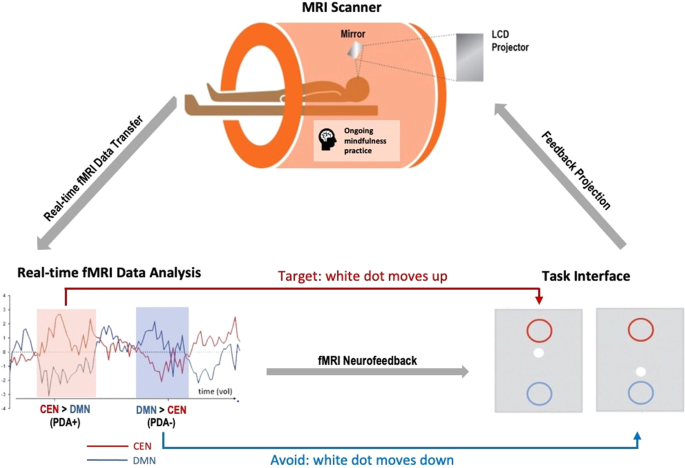This diagram illustrates the process of information transmission to and from an MRI scanner. At the top of the image, the label "MRI scanner" is prominently displayed. Below this, there is a digitally created, translucent orange cylinder representing the MRI scanner, inside which a diagram of a person laying on a bed can be seen. The person's head aligns with a small rectangle that reads "ongoing mindfulness practice." Inside the MRI scanner, a mirror or LCD projector is indicated. 

From the feet of the person, there is a gray arrow pointing diagonally downward to the lower left corner, labeled "real-time fMRI data transfer." Opposite this, on the right side of the diagram, an upward arrow points back towards the MRI scanner, labeled "feedback projection." Below these arrows, in the bottom half of the image, there are graphs labeled "real-time data analysis" and "task interface." The diagrams and arrows collaboratively depict the pathways for real-time data flow and analysis within the MRI neurofeedback loop.